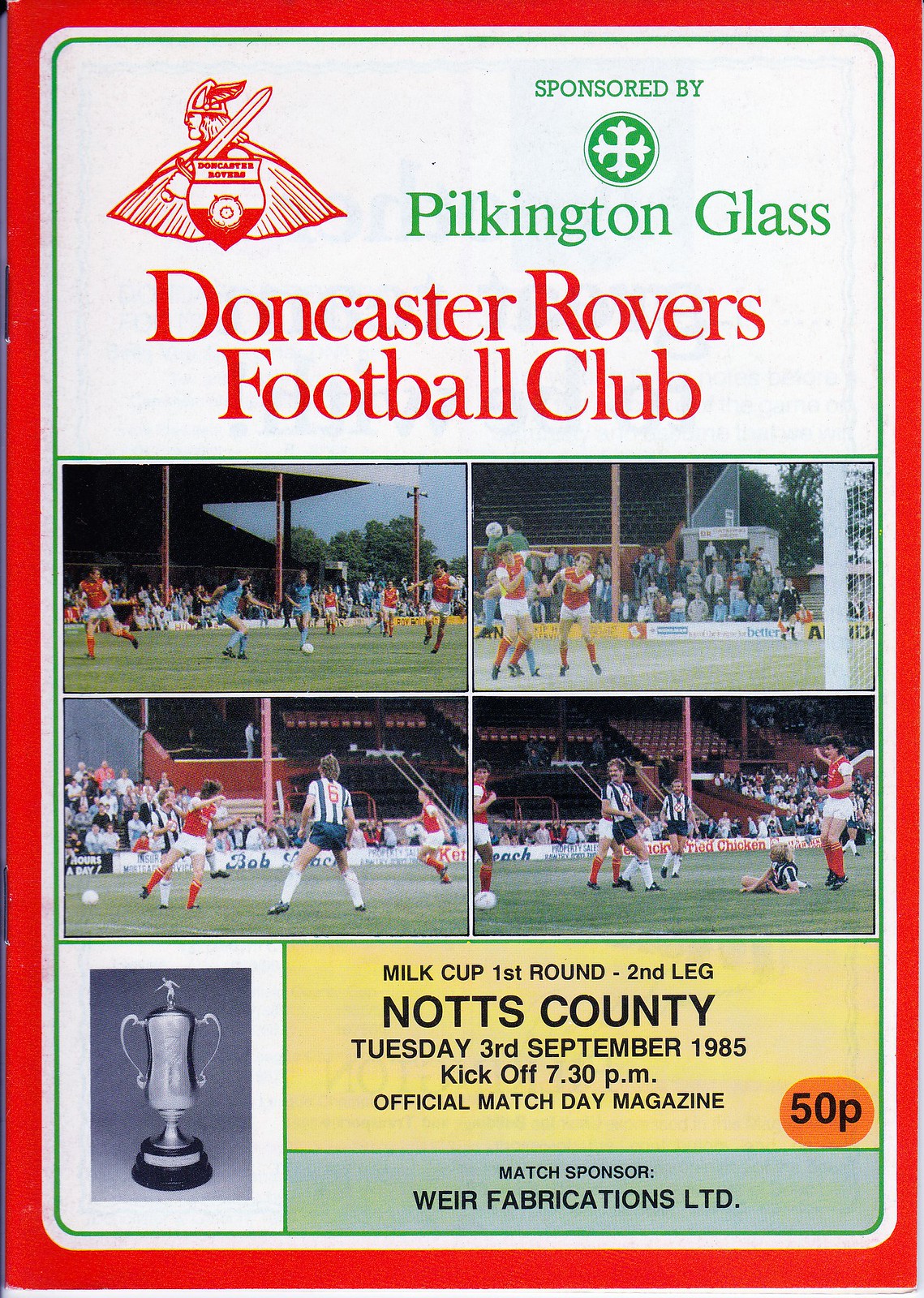The cover of this game day program, or magazine, is a tall rectangular image framed with a bright red border, followed by a white border with curved corners, and an inner green line. At the top, it reads "Sponsored by Pilkington Glass" in green text, accompanied by a circular logo resembling an engraved cross. To the left of the logo, there is a red depiction of a Viking with a sword and shield. Below this, in bold red font, it reads "Doncaster Rovers Football Club." Further down, a grid of four images showcases people playing soccer. Beneath these images, there is a prominent yellow rectangle containing text that reads: "Milk Cup, First Round, Second Leg, Knotts County, Tuesday 3rd September 1985, kickoff 7.30pm, official match day magazine." In the bottom right of this yellow area, an orange oval states "50p." Additionally, a green box near the bottom reads "Match Sponsor Wear Fabrics Ltd." in black text. On the far left, you can see the two staples binding the spine of the booklet.